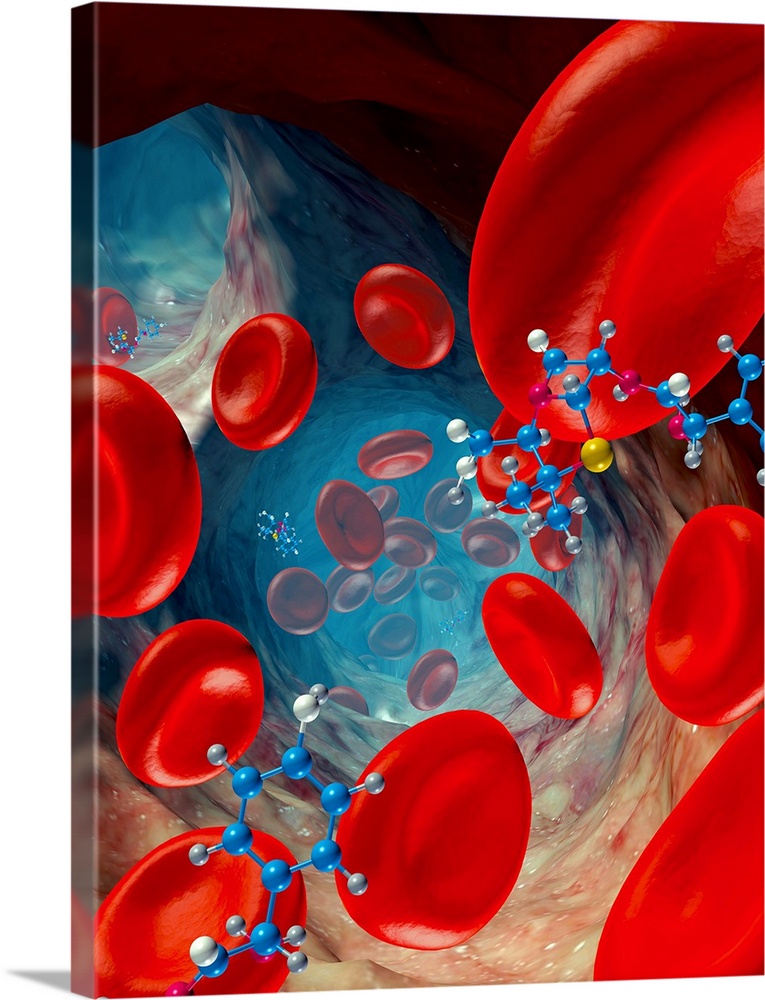This highly detailed, stylized illustration depicts the inside of blood vessels filled with enormous red blood cells. These cells dominate the view as they travel through a cavernous, tube-like structure indicative of a magnified bloodstream. Scattered among the blood cells are intricate molecular structures, resembling DNA or various molecules, composed of interconnected balls and rods forming geometric shapes. The molecules exhibit a spectrum of colors, including blue, white, red, gray, and occasional hints of yellow. The artwork uses perspective and depth, transitioning to a bluish hue in the background, to convey the motion and flow of the blood cells and molecules as they navigate through bifurcated blood vessel paths, one prominently in the center and another in the top left.